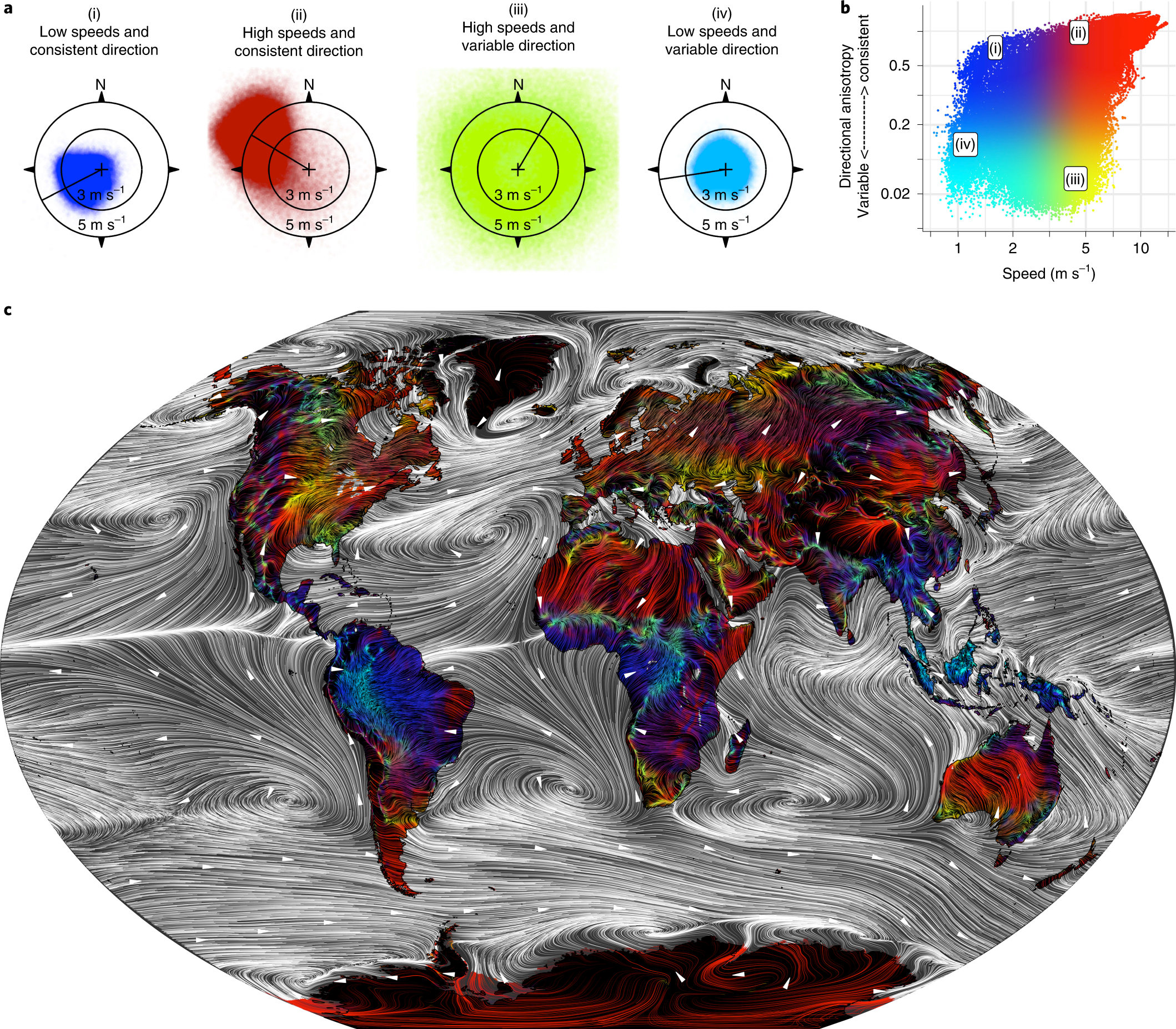This illustration features a stylized, oval-shaped map of the world with the top and bottom flattened. The oceans are depicted with marbled black, white, and gray patterns, while the continents are rendered in a vibrant rainbow of colors, including green, red, orange, blue, yellow, black, and purple. A large red spot is noticeable at the bottom of the image.

At the top of the map, there's a legend with concentric circles in different colors, each representing different weather patterns. The legend details the following: 
1. Low speeds and consistent direction, depicted in blue.
2. High speeds and consistent direction, depicted in red.
3. High speeds and variable direction, depicted in green.
4. Low speeds and variable direction, depicted in light blue.

On the right side of the illustration, a graph labeled "Directional Anisotropy" displays a double-sided arrow between the terms "variable" and "consistent," indicating variability in direction. This graph also features various colors to denote different speed metrics, potentially shown in milliseconds.